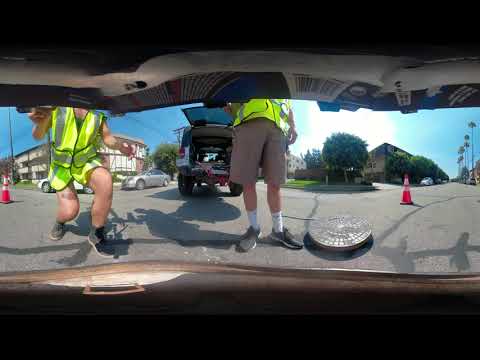This photograph, taken from within a slightly ajar car trunk, captures a unique, panoramic street scene with two men in fluorescent yellow safety vests and khaki shorts. The image angle gives a sense of peering out from inside a vehicle, adding an interesting perspective. The man on the left, slightly bent over, is visible from the shoulders down, showcasing his bare legs, white socks, and dark shoes. The man on the right stands upright, mirroring the attire of the first man. Both men are located near an ajar manhole cover situated on the roadway. In the background, behind the standing man, a truck or SUV with an open rear hatch is visible, displaying some equipment. To the left and right edges of the image, red emergency cones are strategically placed on the road. Additionally, to the far left, you can see a white and a grey car parked near a building with reddish and white paint, surrounded by patches of green grass. In the distant background to the right, a row of palm trees and more residential buildings are visible, grounding the scene in a neighborhood setting.